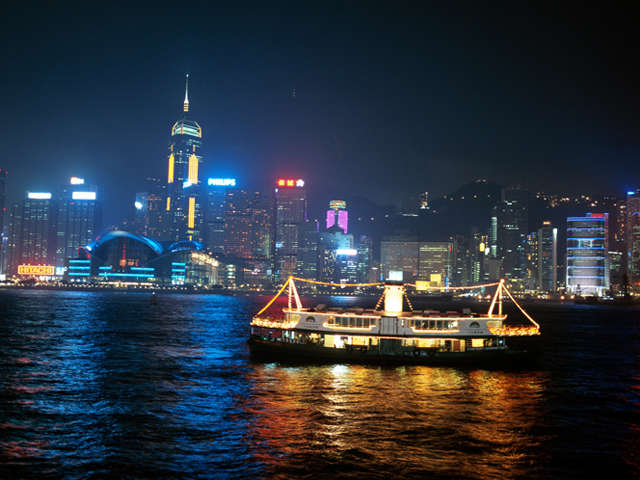This nighttime scene captures a vibrant city skyline, potentially Hong Kong or another Asian city, as evidenced by the Asian writing on several buildings. The city's high-rise buildings are adorned with an array of colorful lights in blue, yellow, green, pink, and red, creating a mesmerizing reflection across the dark waters of the river or ocean. Notably, a large two-tier ferry glows with yellow lights, bathing the surrounding water in warm hues of orange and red. The ferry's top deck is white, while the lower half appears to be green or black. Prominent landmarks in the cityscape include a building with a red Hitachi sign on the left, and another high-rise with a blue and white "Philips" sign. A distinctive event building, perhaps an opera house or theater, stands out with its neon blue lights. Additionally, a tall skyscraper features wide yellow stripes, and another building sports a striking combination of pink and green lights at its peak. The skyline and water are beautifully illuminated by the myriad of city lights, creating a stunning and picturesque nocturnal view.